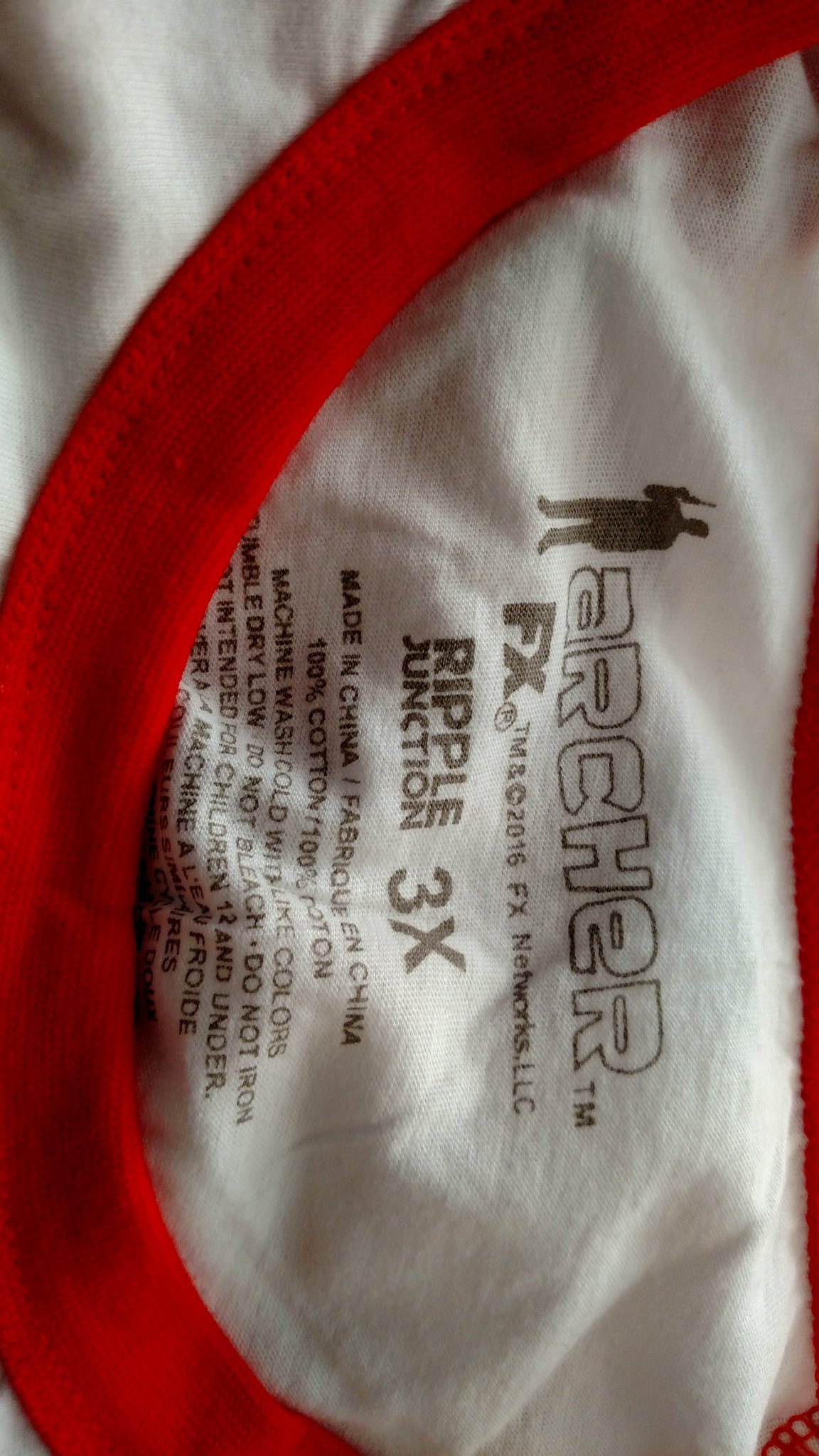A vertically oriented close-up image of a shirt label integrated into the fabric, rather than a separate tag. The text is aligned sideways, making it slightly challenging to read. The label features a small silhouette of a man holding a gun, with the word "Archer" beside it, indicative of the FX TV show. Below that, it reads "FX TM © 2016 FX Networks LLC," followed by the manufacturer "Ripple Junction" and the size "3X." Additional text includes "Made in China," "100% Cotton," and laundry instructions, though some details are obscured due to the angled perspective. The shirt fabric colors visible in the image are red and white.